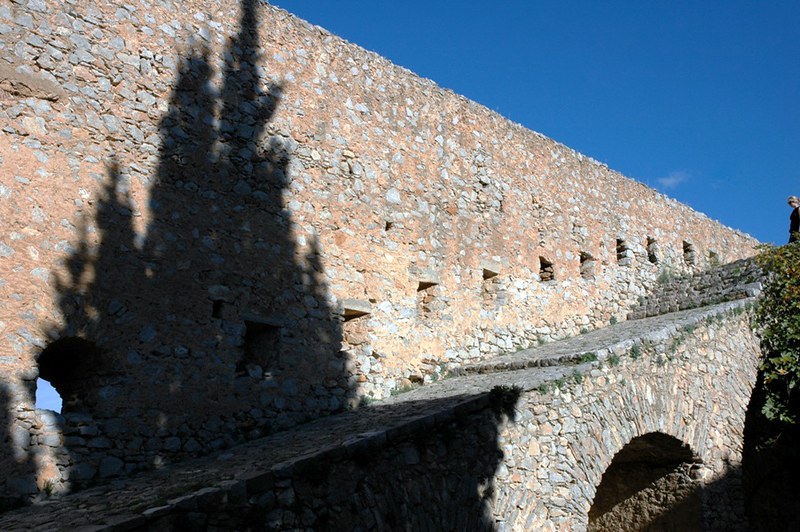This photograph captures an ancient stone pathway leading up to a high wall, reminiscent of castle ruins, possibly part of a historic fortification. The pathway, composed of aged masonry with irregular stones, ascends gently and features arches that appear to lengthen as they rise. A lone figure, dressed in black, stands at the top of the steps, adding scale to the imposing structure. Shadows from a nearby large pine tree stretch across the stone wall, accentuating the height and depth of the scene, while a more deciduous tree can be glimpsed on the right side of the image.

Along the walkway, windows or slotted openings can be seen, designed perhaps for ancient defenders to survey or protect against intruders. The medieval aesthetic is further enhanced by the worn, mossy stones mixing with patches of light brownish-red hues. The sky above is clear and blue, offering a serene backdrop to the rugged, historical edifice. This site, likely a popular tourist destination for history enthusiasts, exudes a timeless quality and speaks of its storied past.